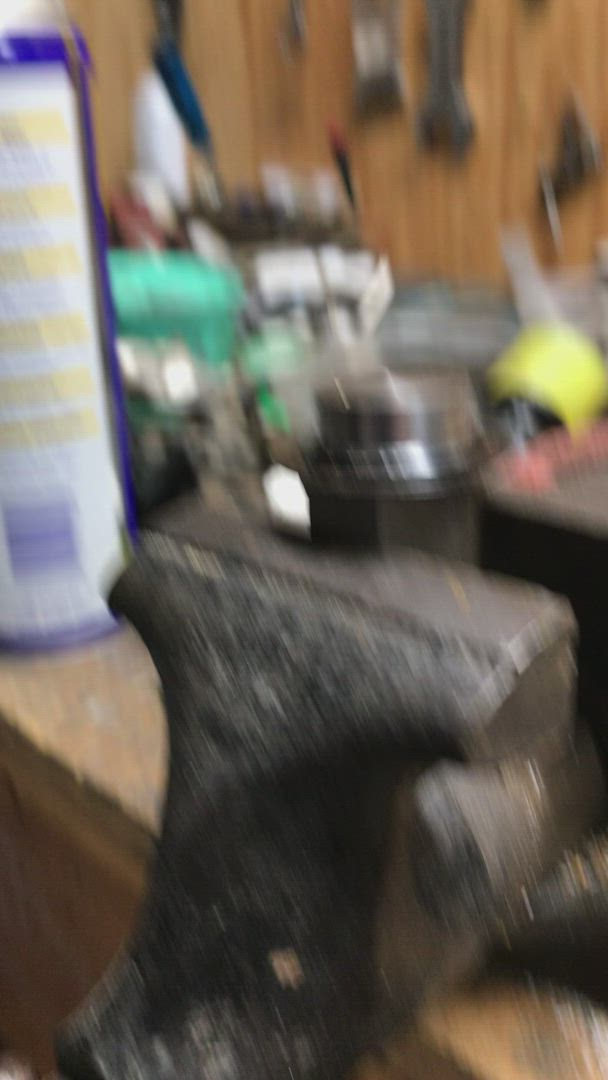The photograph is a very out-of-focus image depicting a cluttered workshop. Dominating the foreground is a large cast iron vise with a handle, potentially holding a dual-toned (dull and shiny silver) piece of metal. To the left of the vise, there is a colorful container, likely a purple spray can of chemical or lubricant, featuring a prominent white label with yellow markings and possibly a barcode. The background showcases a wooden wall adorned with various tools hanging, resembling a pegboard setup typical of a mechanic's workspace. Scattered across the concrete-topped workbench are a variety of objects including green and blue bottles, and equipment parts with hues of yellow and silver, contributing to the overall sense of disarray in the workshop.